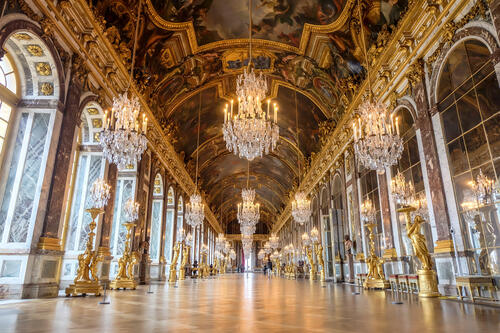The image depicts an opulent and grandiose indoor scene reminiscent of a European palace, potentially the Hall of Mirrors at the Palace of Versailles. The central perspective focuses on a long, majestic hallway adorned with lavish decorations. On the right side of the hallway, tall, arched windows allow bright daylight to flood in, while on the left, arched windows and mirrors contribute to an airy, expansive feel. Each window is flanked by elegant golden statues, positioned beside brown marble pillars add to the regal ambiance.

The floor is smooth and reflective, likely made of polished wood or white tile, enhancing the room's spaciousness by mirroring the intricate details from above. Overhead, an arched vaulted ceiling commands attention, subdivided into panels housing ornate, allegorical, and naturalistic paintings, each bordered with ornate golden trim. Below these paintings, the ceiling's edges are embellished with luxurious golden crown moldings.

Hanging from the ceiling, grand crystal chandeliers with candle lights add a touch of glittering sophistication. These chandeliers are spaced in rows, extending further down the hallway, contributing to the hallway's continuous splendor. The overall composition of the hall with its gleaming statues, opulent decorations, and the interplay of natural light creates a captivating, royal atmosphere, highlighting the architectural magnificence and artistic richness of this palace interior.